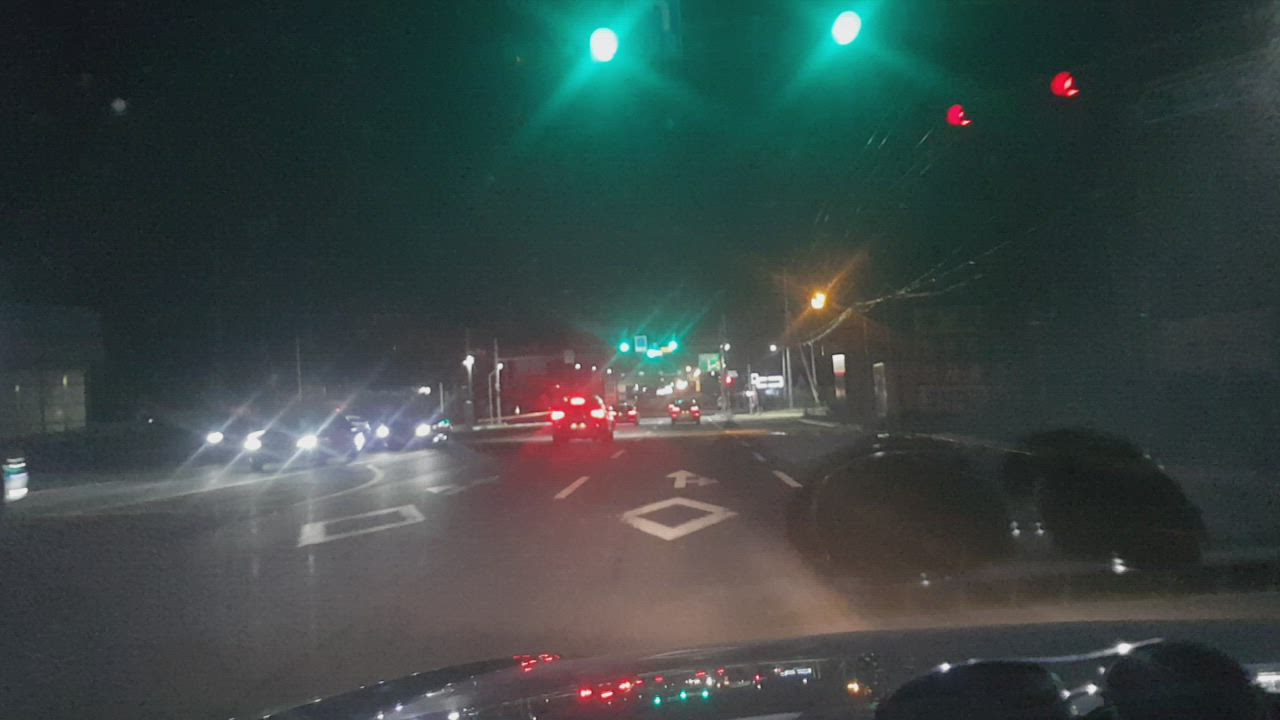This captivating nighttime photograph, captured in landscape orientation, offers a unique perspective through the front windshield of a car in motion. At the bottom of the frame, a pair of sunglasses rests on the dashboard, their presence doubled by a reflection in the windshield overhead. The scene outside is enveloped in darkness, illuminated by two green traffic lights at the top of the image, signaling through the night. Ahead, a few cars with glowing red taillights cruise down the freeway, while to the left, the headlights of oncoming traffic streak through the night. The composition beautifully intertwines elements of the interior and exterior, capturing the essence of a nocturnal journey.